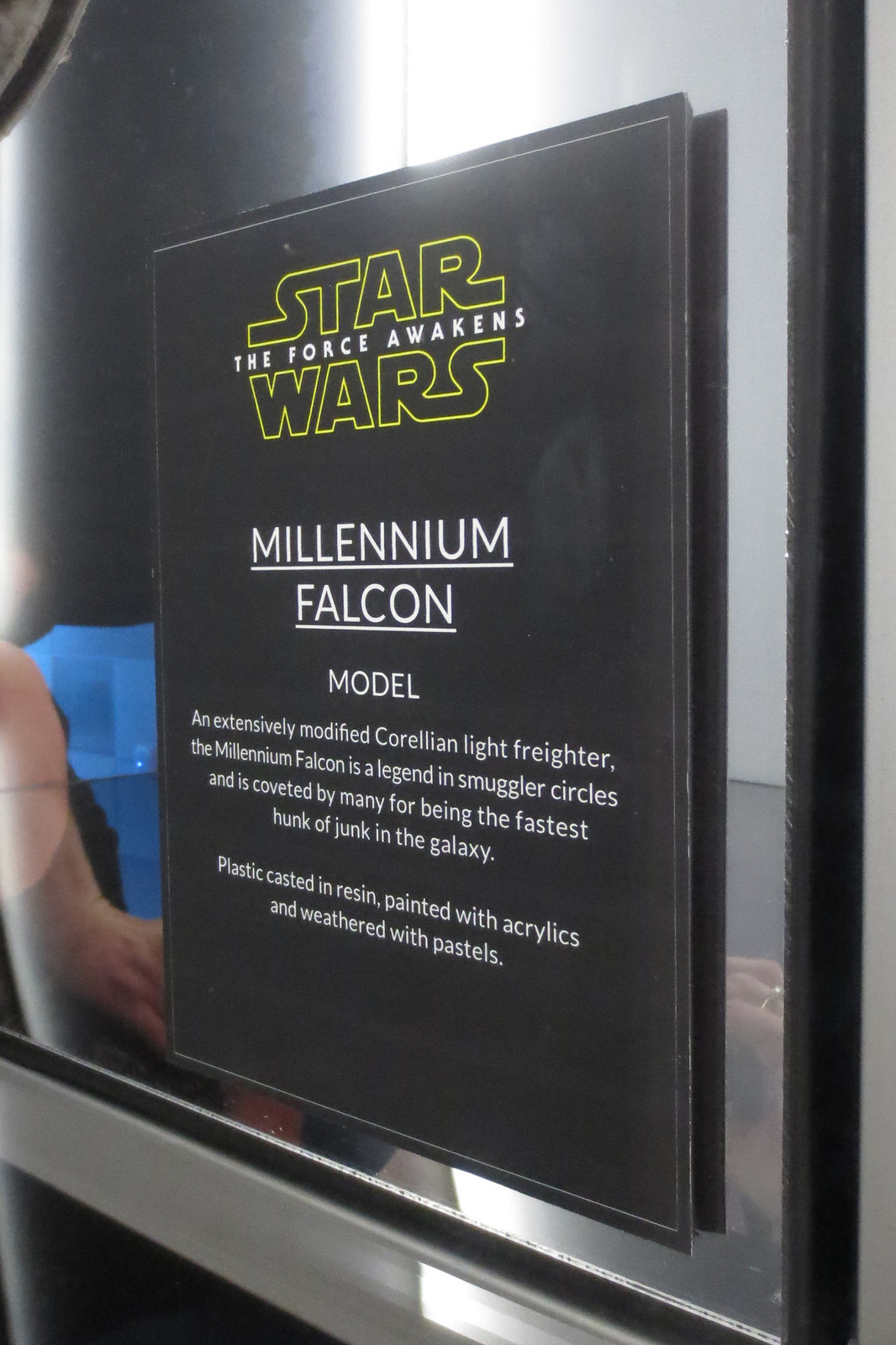The photograph captures a detailed, side-angled view of a rectangular black sign with a mirrored background, possibly mounted on a reflective surface. The sign prominently features the iconic Star Wars logo at the top, outlined in yellow. Below this, in white text between the words "Star" and "Wars," it states "The Force Awakens." Further down, the sign provides information about the Millennium Falcon, describing it as "an extensively modified Corellian light freighter" and "a legend in smuggler circles," coveted for being the "fastest hunk of junk in the galaxy." The text is presented in white and includes underlined headings for clarity. The sign itself is crafted with meticulous detail, cast in resin, painted with acrylics, and weathered with pastels, lending it an authentic and rugged appearance. In the background, another picture or a reflection can be seen, along with the faint outline of a person's arm in the bottom right corner, adding an element of depth to the image.